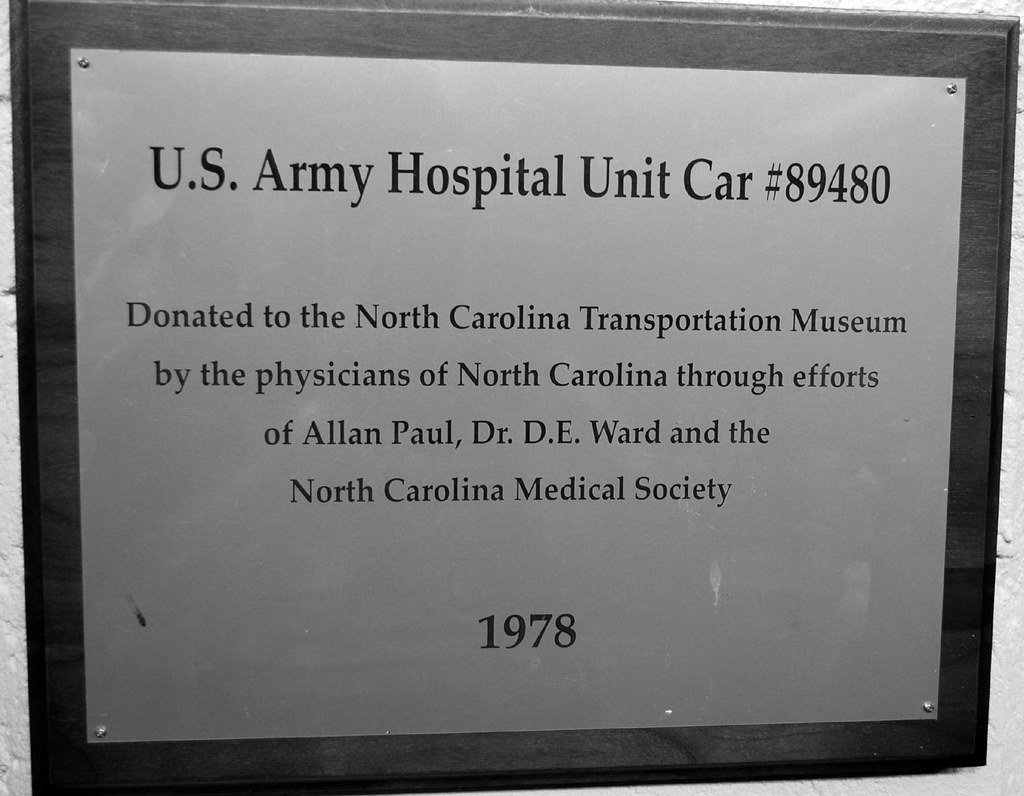The image shows a close-up of a detailed plaque mounted on a wall. The plaque is framed in dark gray or black wood with a protective glass cover. Inside the frame, a metallic-looking sheet, possibly brass, is affixed with screws at each corner. The surface of this sheet is adorned with black text that reads: "U.S. Army Hospital Unit Car No. 89480. Donated to the North Carolina Transportation Museum by the Physicians of North Carolina through efforts of Alan Paul, Dr. D.E. Ward, and the North Carolina Medical Society, 1978." The plaque appears to have some signs of wear, including a few scuffs and possible fingerprint marks. Overall, it commemorates the donation of a hospital unit car by North Carolina physicians in 1978.